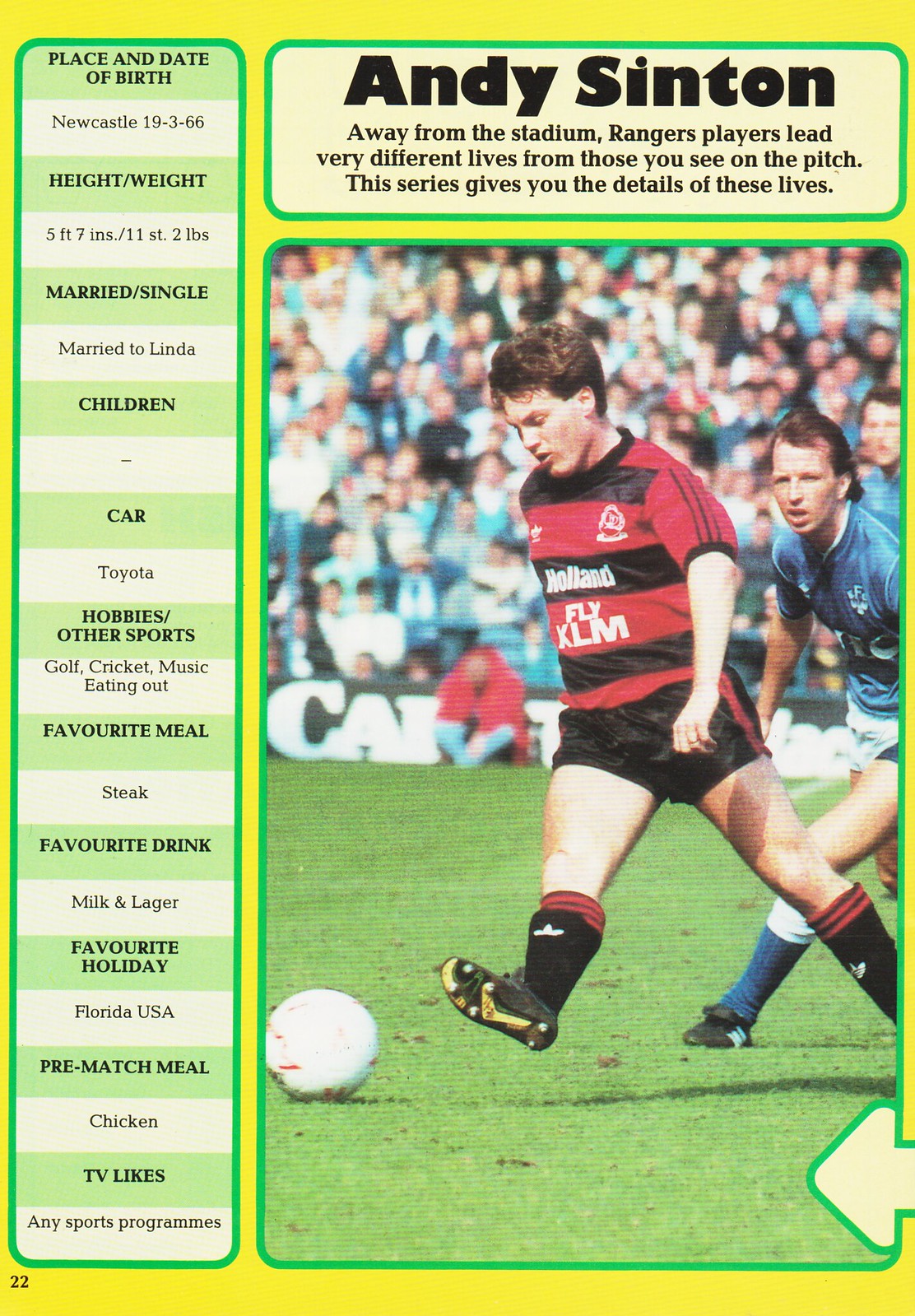This image, which appears to be an older photo likely from a 1993 magazine, features a character profile for soccer player Andy Sinton. The background of the page is predominantly yellow with three distinct boxes. The left box details Andy Sinton's personal statistics, including his place of birth (Newcastle), height (5 feet 7 inches), weight (11 stone, 2 pounds), marital status (married to Linda), car (Toyota), and hobbies (golf, cricket, music, and dining out). His favorite meal is steak, favorite drink is lager, and favorite holiday destination is Florida, USA. Additionally, it mentions his pre-match meal is chicken, and his TV preferences are any sports programs. The text in the top right box emphasizes that Rangers players, like Andy, lead very different lives away from the stadium, offering insights into those lives. The large bottom right photo shows Andy Sinton, a white man with brown hair, wearing a red and black jersey and black shoes, running and about to kick a soccer ball. The image has an older, faded quality typical of 1990s photo development.